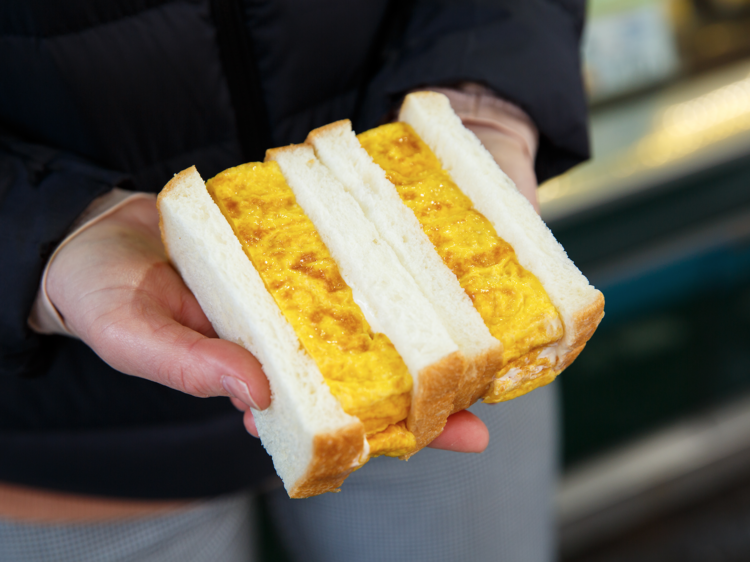In this color photograph, a person is holding two halves of a simple egg sandwich in their hand. Each sandwich features slices of white bread filled with a yellow, golden brown egg mixture, which appears to be about an inch thick. The bread is moist with visible crusts on the sides but not on the top or bottom. The person holding the sandwiches wears a dark-colored long-sleeved shirt with a pink layer underneath, along with light blue jeans. The background is out of focus, suggesting an indoor setting with a counter and a bar area. Colors in the photo include black, pink, light blue, yellow, golden brown, and white, with an indistinct possible green tinge and a barely discernible sign in the upper right.